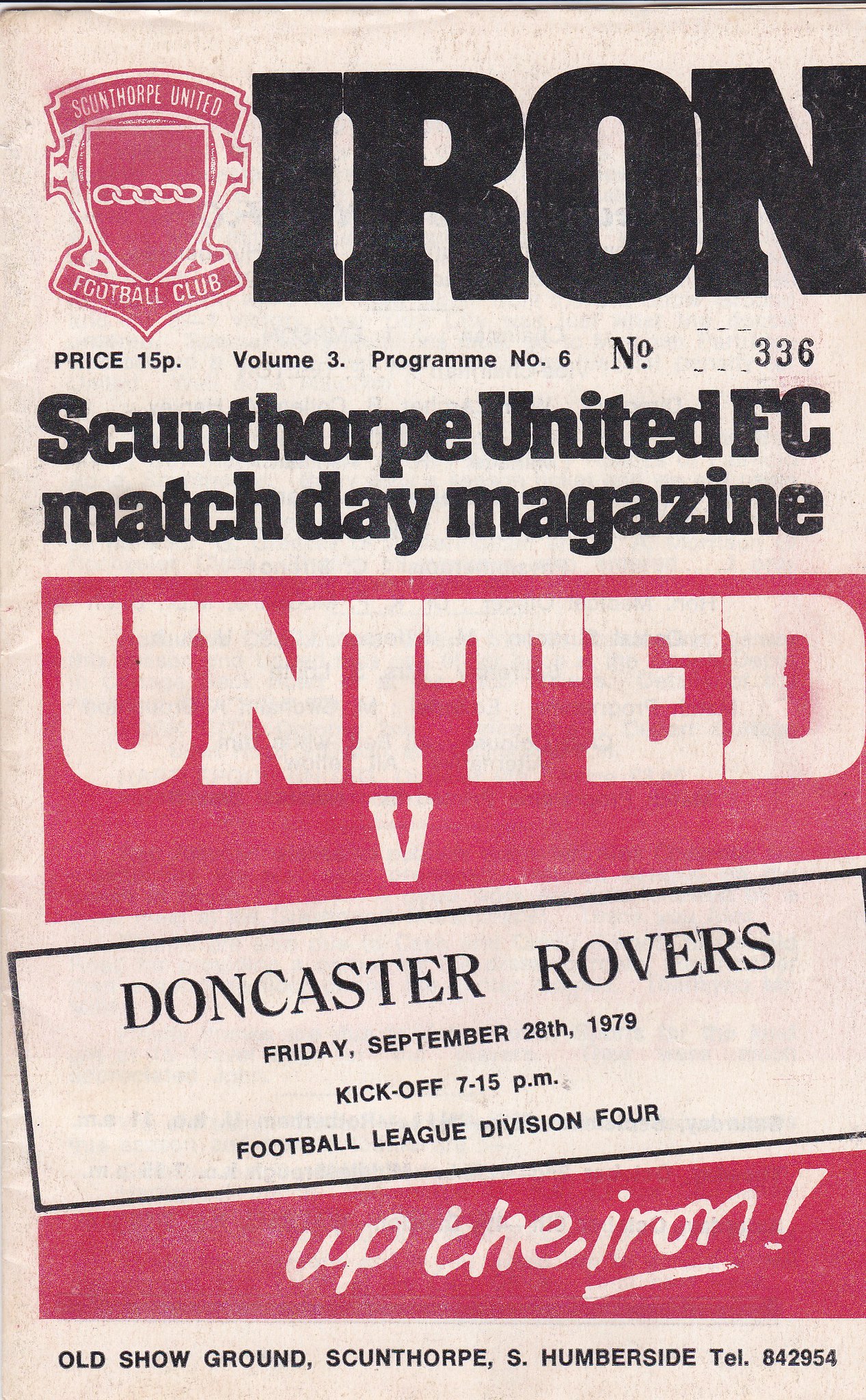The front cover of the vintage sports magazine, titled *Iron in Black*, highlights Scunthorpe United Football Club's match day against Doncaster Rovers. Priced at 15 pence, this edition is Volume 3, Program No. 6, and No. 336. In the top left corner, the Scunthorpe United FC logo, featuring a shield with five interconnected links, is displayed. Adjacent to the logo, in black text, it reads "Iron". Below, the text details: *Scunthorpe United FC Match Day Magazine, United v Doncaster Rovers, Friday September 28, 1979, Kickoff 7.15 PM, Football League Division 4*. The cover transitions into a maroon box with white text proclaiming *Up the Iron!*. The bottom segment, set in black text, gives the location as *Old Showground, Scunthorpe South, Humberside* with the contact number *842-954*. The overall aesthetic of the cover is distinctly vintage, with a beige-white paper background and a mix of black and maroon text for high contrast.